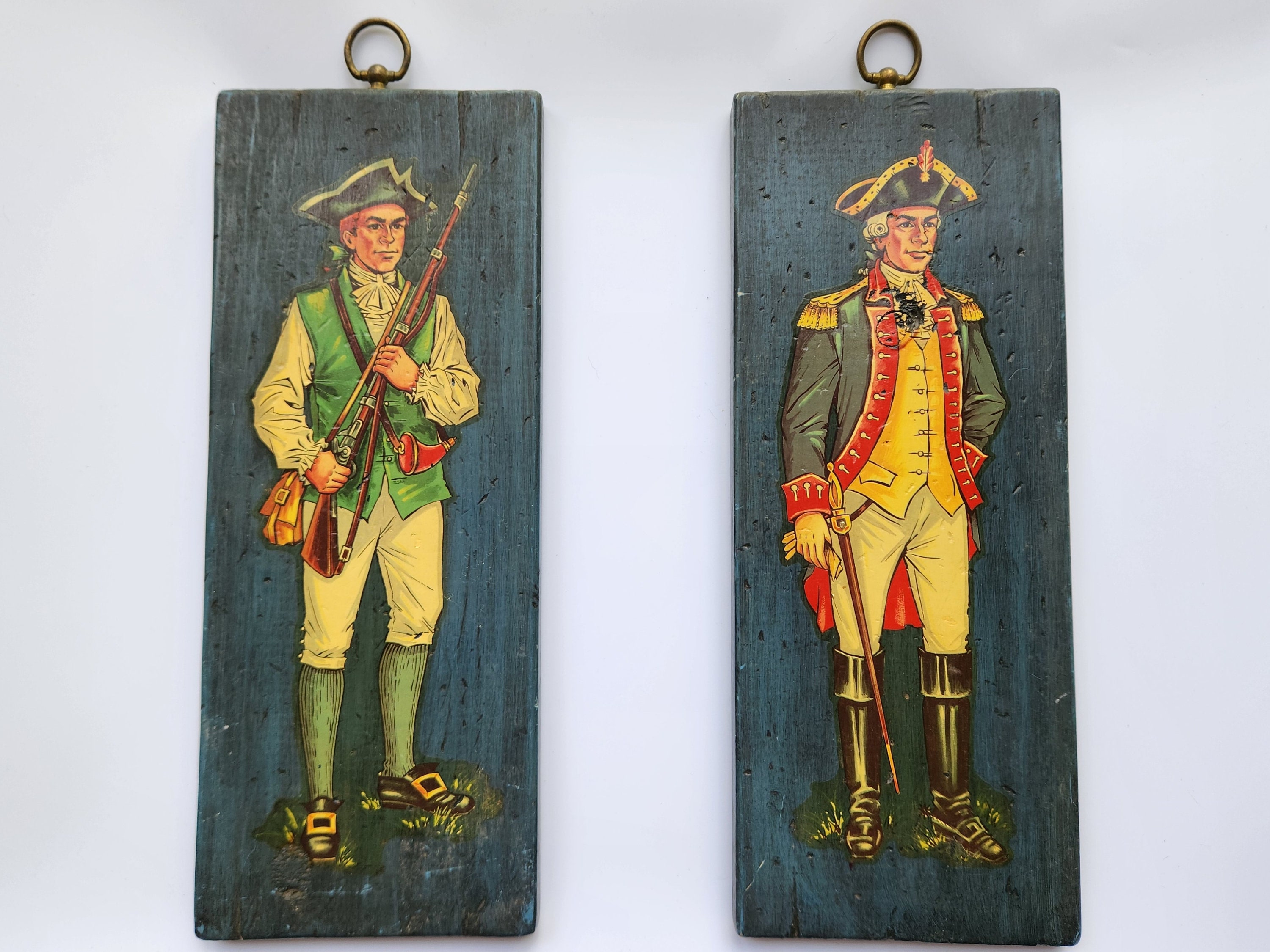The image depicts two rectangular, painted wooden slates, each featuring a historical soldier against a dark blue or blue-gray background. Both slates are equipped with brass loop hooks at the top for hanging.

The soldier on the left is portrayed in a green waistcoat with a white shirt, knee-length white trousers, and long green socks. He is wearing black, low-cut shoes adorned with square gold buckles. His hat is simpler in design compared to the other soldier's. He wields an old-style musket with a bayonet attached to the front and also carries a mustard-colored side bag slung across his chest. Additionally, he has a horn at his left hip, possibly for gunpowder or signaling.

In contrast, the soldier on the right is characterized by his higher rank, evidenced by a black hat with gold trim and a decorative flower, indicative of a captain or officer. He has white hair styled in curls, possibly a wig. His attire includes a yellow waistcoat under a dark-colored coat trimmed with gold braids and red lapels, which also features long tails. He wears knee-length black boots, white trousers, and gloves, and is equipped with a sword at his right hip.

Both soldiers exhibit detailed attire, suggesting their roles in ancient English military, with the soldier on the right displaying more elaborate and mature characteristics. These tasteful, historical renderings on wooden slates serve as decorative items, ideal for adding a touch of vintage military aesthetics to a home.